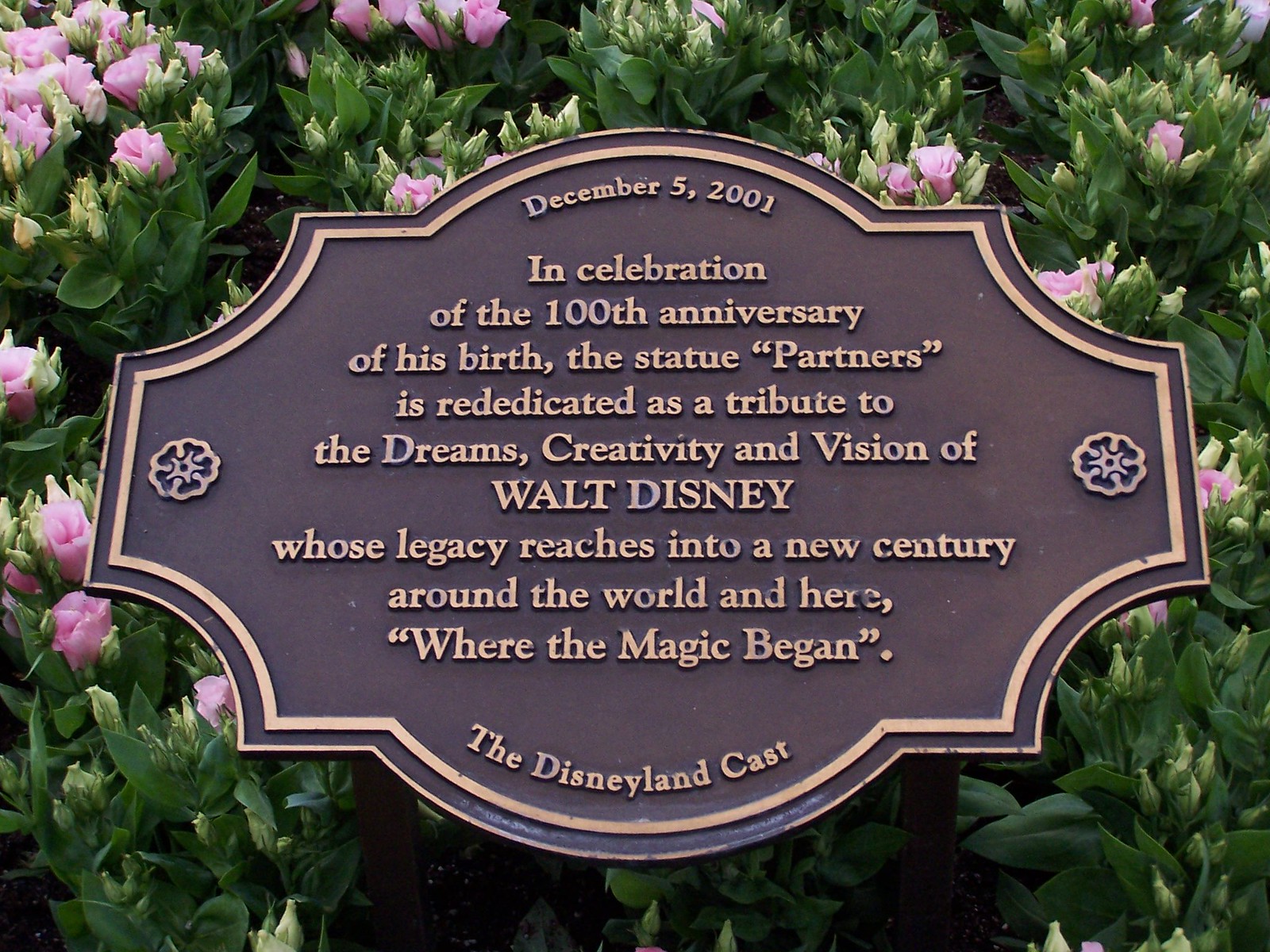The photograph depicts a pristinely maintained memorial plaque at Disneyland, surrounded by vibrant, pink flowers that resemble tulips, nestled among lush green leaves and dark soil. The plaque, with a bronze-like finish and gold lettering, commemorates the rededication of the statue "Partners" on December 5, 2001. This rededication marks the 100th anniversary of Walt Disney's birth, honoring his dreams, creativity, and vision. The inscription emphasizes Walt Disney's enduring legacy, which continues to inspire new generations both worldwide and at the birthplace of Disney magic. The plaque's unique design includes a copper border and floral engravings on either side, contributing to its elegant appearance amidst the natural floral backdrop.